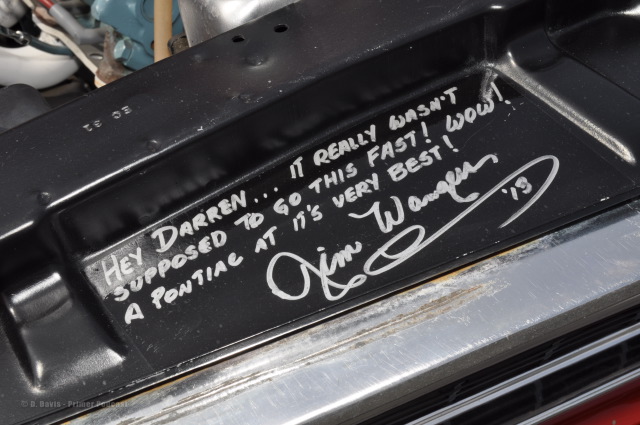This photograph captures a close-up shot of what appears to be an interior component of a vehicle, depicted against a stark black background. Dominating the forefront is a sleek, silver section, possibly a part of the dashboard or another metallic element within the car. In silver Sharpie, a handwritten message is inscribed on the black surface, reading: “Hey Darren... it really wasn’t supposed to go this fast! Wow! A Pontiac at its very best!” Accompanying this enthusiastic note is a sizable signature, seemingly from someone named "Jim," with the last name beginning with 'W'—potentially Wagner. Beneath the signature is an artistic swirl, within which the number 13 is inscribed, adding a unique and personal touch to the message.